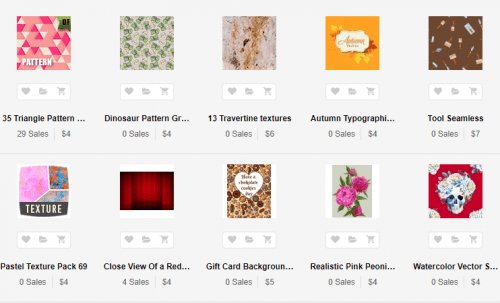The image features a vibrant assortment of detailed patterns and textures arranged in a grid format. In the top left, a pink square showcases 25 intricate triangle patterns, set meticulously in 25 groups. Adjacent to it, a green square presents a delicate Damascus design, finely detailed and ornate. Below, a brown square is etched with text in a travertine style, numbering 13 distinct texts. An orange square captures attention with its autumn-themed "grider" pattern, rich in warm hues.

Continuing, another brown square is embellished with a sprinkles-like texture, intersected by two seams, and interspersed with listed contents. Further along, a pink square offers a varied panel texture pack. To the right, red curtains frame a segment titled “Chinese View,” featuring a deep, vivid red.

A heart shape outlines the centerpiece, encircled by peanuts, set against a gift card backdrop adorned with realistic pink flowers. On a personal note, a red square depicts a white skull wearing a top hat, a stark contrast against its vibrant backdrop, and is labeled as "white color victor."